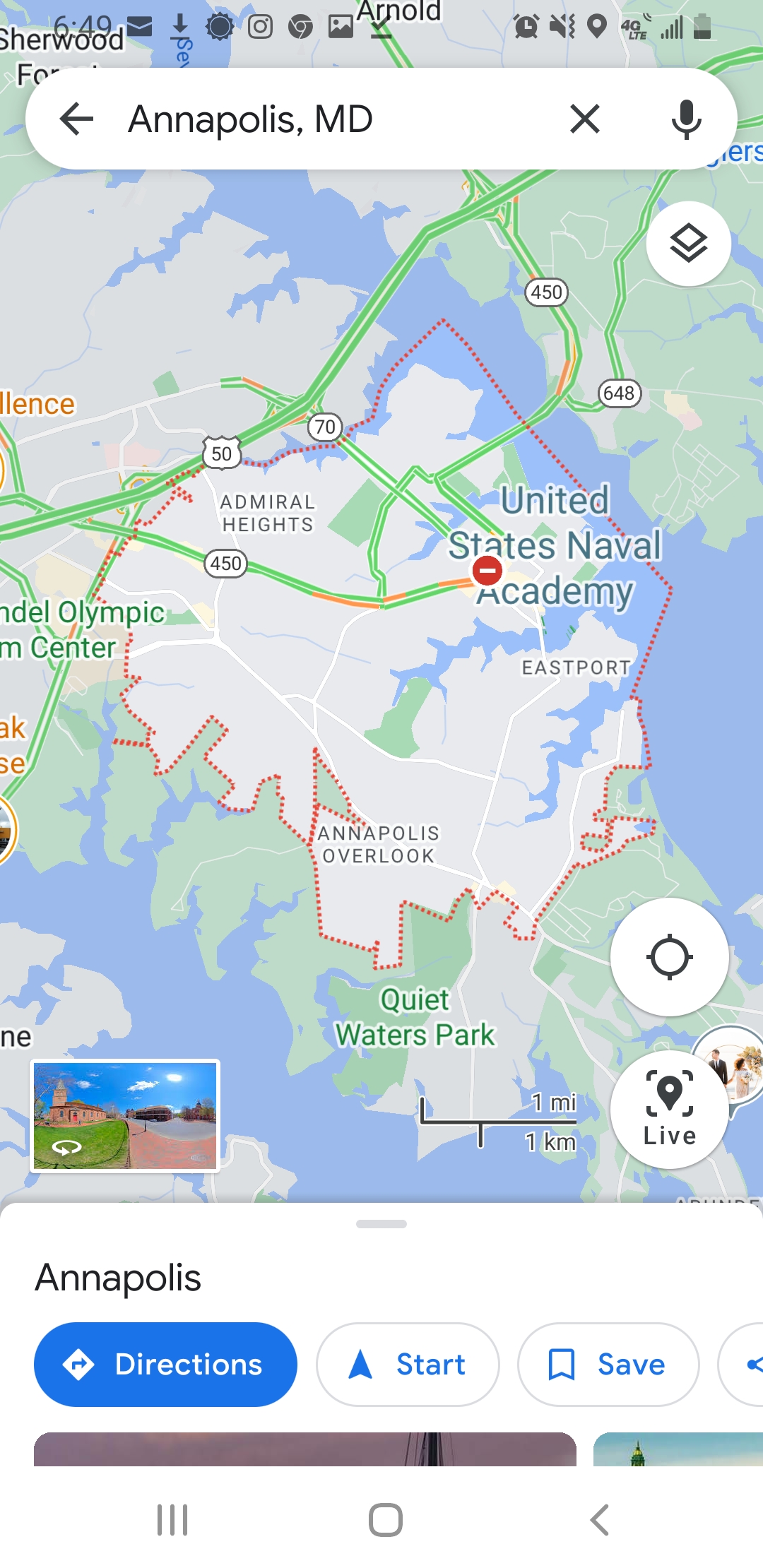This image showcases a screenshot from a mobile map application. Dominating the screen is a map displaying the area around Annapolis, MD, rendered in blue, gray, and green hues to differentiate various terrains and structures. At the top, there's a search bar reading "Annapolis, MD," accompanied by an 'X' icon for clearing the search and a microphone icon for voice input. 

A circular white button on the interface allows users to adjust the zoom level of the map. A Google Maps-style street view thumbnail occupies the bottom left corner, providing a ground-level perspective of the area. In the bottom right, a button labeled "ALIVE" lets users mark or ping specific locations on the map.

Highlighted directions to Annapolis are prominently displayed in blue, guiding the viewer along a specified route. Below the map, three unselected white buttons with blue text offer additional functionalities: "Start" to begin navigation, "Save" to store the route for future reference, and "Share" to distribute the directions to others.